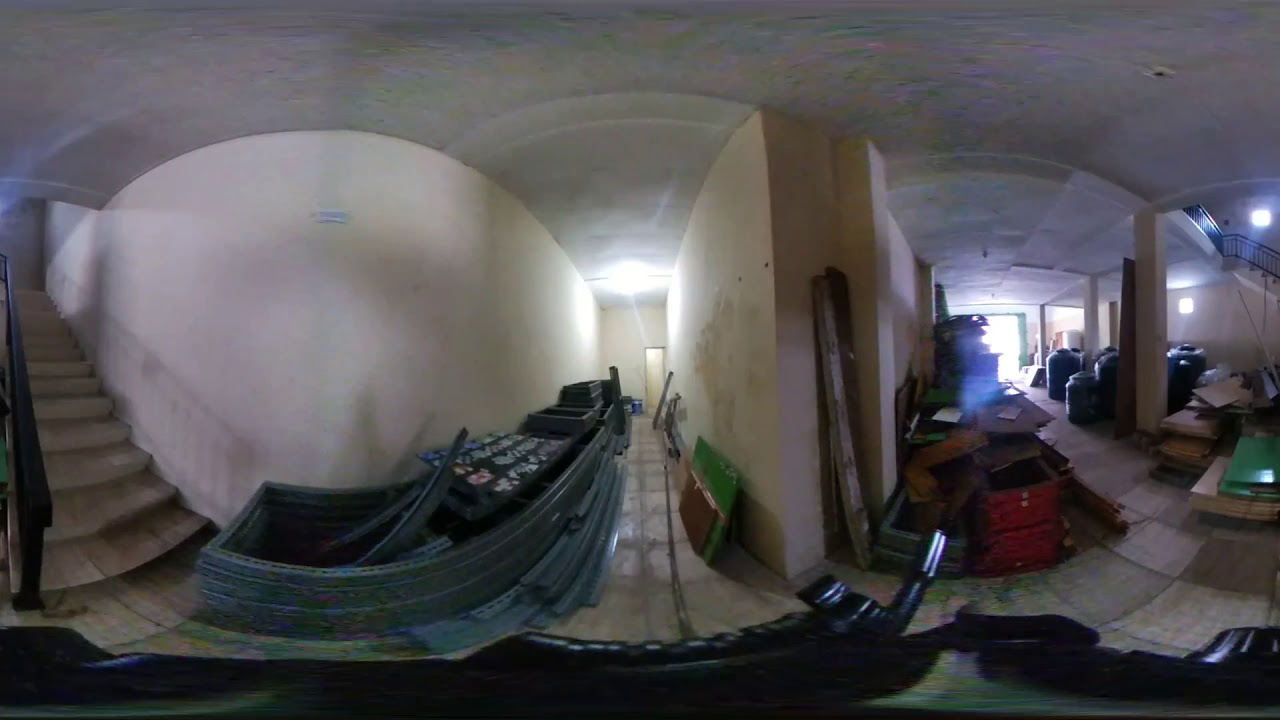The image appears to be taken with a wide-angle lens, causing significant distortion and making it somewhat challenging to interpret the scene accurately. Nevertheless, the setting seems to be a storeroom or possibly a basement storage area with white, curved adobe walls. On the left side of the image, a metal-railed staircase descends, with various containers and items cluttered at its base. Adjacent to the staircase is a small hallway also filled with objects, including long green items stacked atop each other.

In the central part of the storeroom, there are tables that are folded and flipped upside down, stacked on top of each other. Surrounding these tables are wooden planks and possibly additional chairs of different colors, such as green and brown. The corridor divides the room, and along this divider, more flat cardboard boxes and circular bins are visible.

On the right side of the room, multiple metal containers and boxes, including green, red, and brown ones, are lined up along the walls. These boxes are piled high and extend towards the back of the building. There is also a large door on this side, possibly providing access to the outside for moving large items like tables and chairs. The overall visual impression is one of a cluttered and densely packed storage area filled with various types of boxes, containers, and folded furniture.